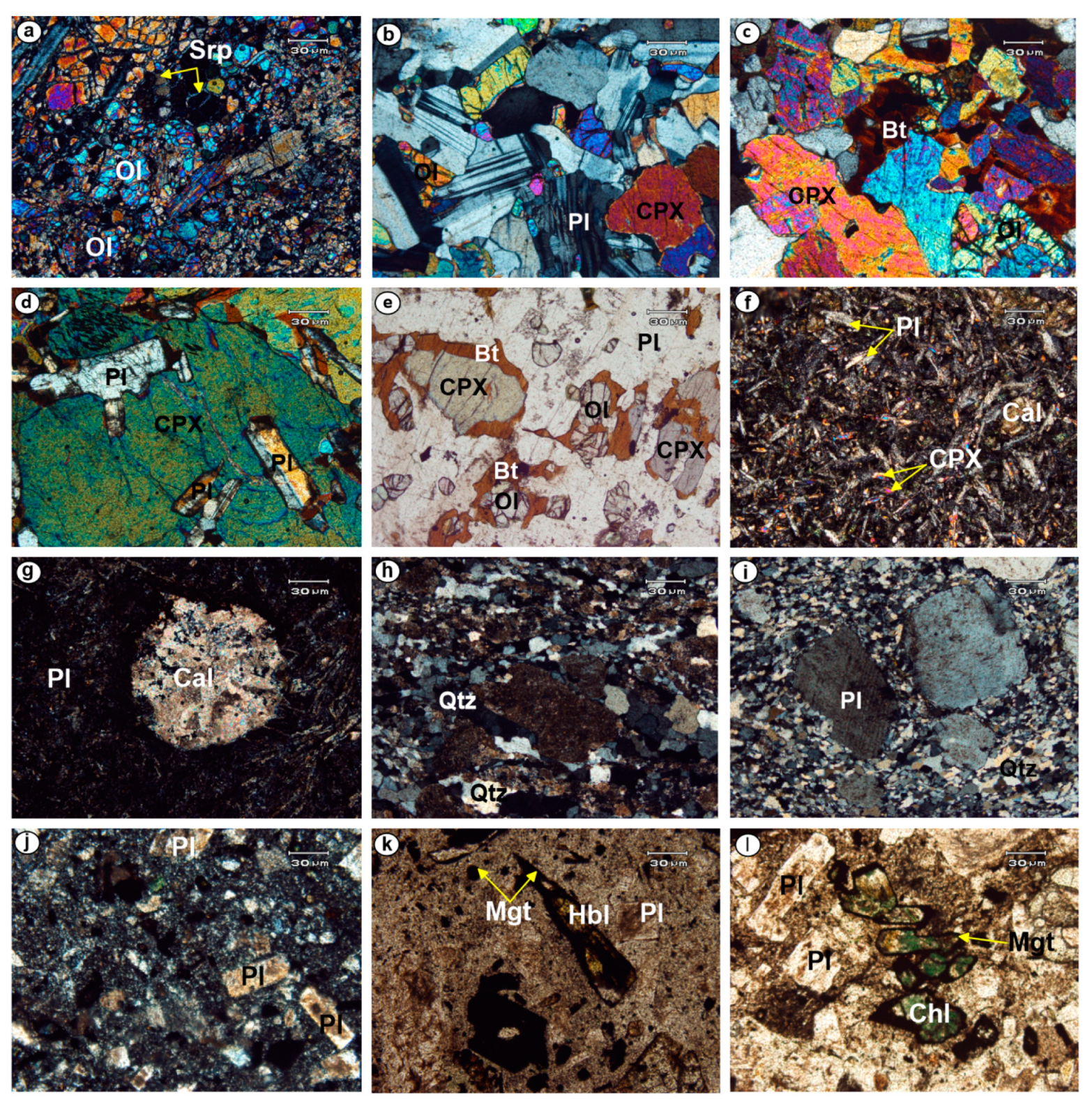The image presents a detailed compilation of 12 microscopic photographs of various minerals or rocks, meticulously arranged in a grid with four rows and three columns. Each photograph, labeled from A to L in the top left corner, captures distinct specimens such as quartz, magnetite, and chlorite at significant magnification, discernible by the micrometer scales provided.

The minerals are rendered in a rich palette of colors including red, pink, purple, brown, teal, black, yellow, green, light green, white, off-white, rust, lime green, and violet, creating a vivid visual spectrum. Each image bears specific symbolic annotations like PI, C-P-X, BT, Q-T-Z, CAL, MGT, HBL, reflecting the natural variety and composition of the specimens. Arrows indicate specific particles within the images, maintaining clarity and precision. The overall setting is bright and clear, suggesting an optimal lighting environment for microscopic imaging, and the clarity of the digitally created images underscores the detailed textures and structures of each mineral sample.